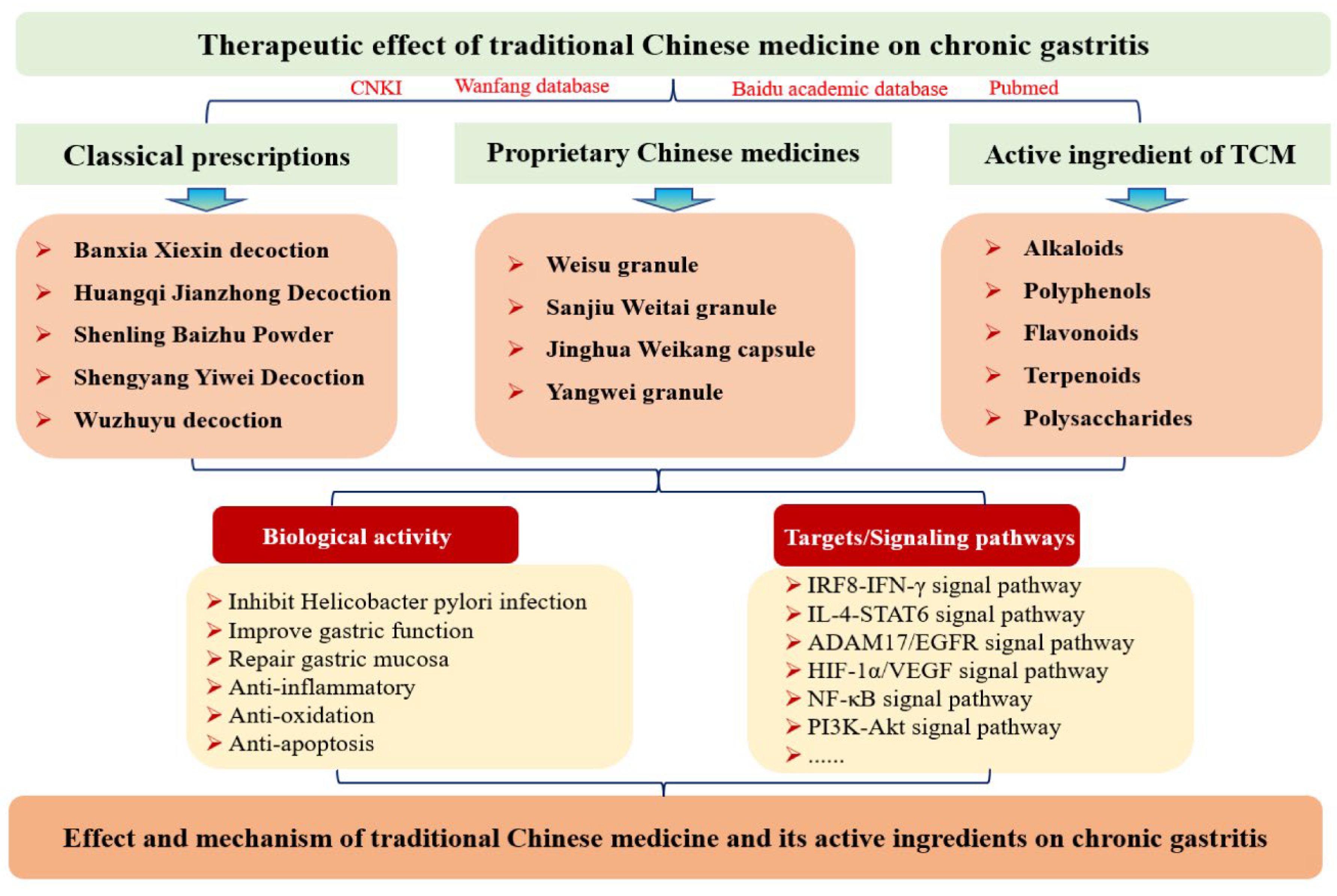The image is a detailed flowchart on a white background, utilizing various colored boxes in light green, tan, orange, and red to visually segment information. It is titled "Therapeutic Effect of Traditional Chinese Medicine on Chronic Gastritis" in black text on a green background at the top. The chart is structured in a genealogical style, with a descending black line that branches out into three primary categories: "Classical Prescriptions," "Proprietary Chinese Medicine," and "Active Ingredient of TCM," each labeled in black on a green background.

Under the "Classical Prescriptions" heading, the flowchart lists specific formulas such as Banxia Xiexin Decoction, Huangqi Jianzhong Decoction, Shenling Baizhu Powder, Shengjiang Xiefei Decoction, and Wumei Decoction. The "Proprietary Chinese Medicine" section includes items like Weisu Granule, Sanjiu Weitai Granule, Jinyizhi Weikang Capsule, and Yangwei Granule. The "Active Ingredient of TCM" category details compounds such as Alkaloids, Polyphenols, Flavonoids, Terpenoids, and Polysaccharides, all highlighted in pale pink or tan boxes with blue arrows pointing downward.

Further down, the flowchart splits into two additional categories: "Biological Activity" and "Target Signaling Pathways," both labeled in red with white text. Under "Biological Activity," it lists actions such as inhibiting Helicobacter pylori infection, improving gastric function, repairing gastric mucosa, anti-inflammatory effects, antioxidation, and anti-apoptosis. "Target Signaling Pathways" includes pathways like NF-κB, PI3K/Akt, IL-4/STAT6, TLR4/MyD88, EGFR, and HIF-1α/VEGF.

At the bottom of the chart, on a tan background with black text, the flowchart concludes with the phrase "Effect and Mechanism of Traditional Chinese Medicine and its Active Ingredients on Chronic Gastritis," a reiteration of the top label, summarizing the therapeutic impacts and mechanisms outlined above.